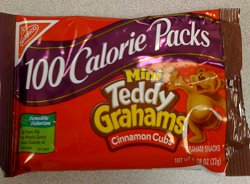This image features an unopened package of Nabisco's Mini Teddy Grahams, specifically the 100-calorie packs of the cinnamon-flavored variety. The packaging is predominantly red, with a vibrant and eye-catching design. The "Mini Teddy Grahams" lettering is prominently displayed, with "Mini" and "Grahams" in yellow letters outlined in brown. The word "Teddy" is written in white. Below this, a small red banner announces the cinnamon flavor.

At the center of the package is an animated depiction of a cheerful teddy bear, which adds a playful and engaging element to the design, distinguishing it from an actual teddy bear. A large banner at the top of the package boldly declares "100 Calorie Packs," emphasizing the product's portion-controlled, diet-friendly appeal. 

The familiar red Nabisco logo is situated in one corner, ensuring brand recognition. In the lower left-hand corner, a green chart provides nutritional information, reinforcing the product's health-conscious marketing message. This detailed and colorful package design is meant to attract health-minded consumers, especially those seeking low-calorie snacking options.